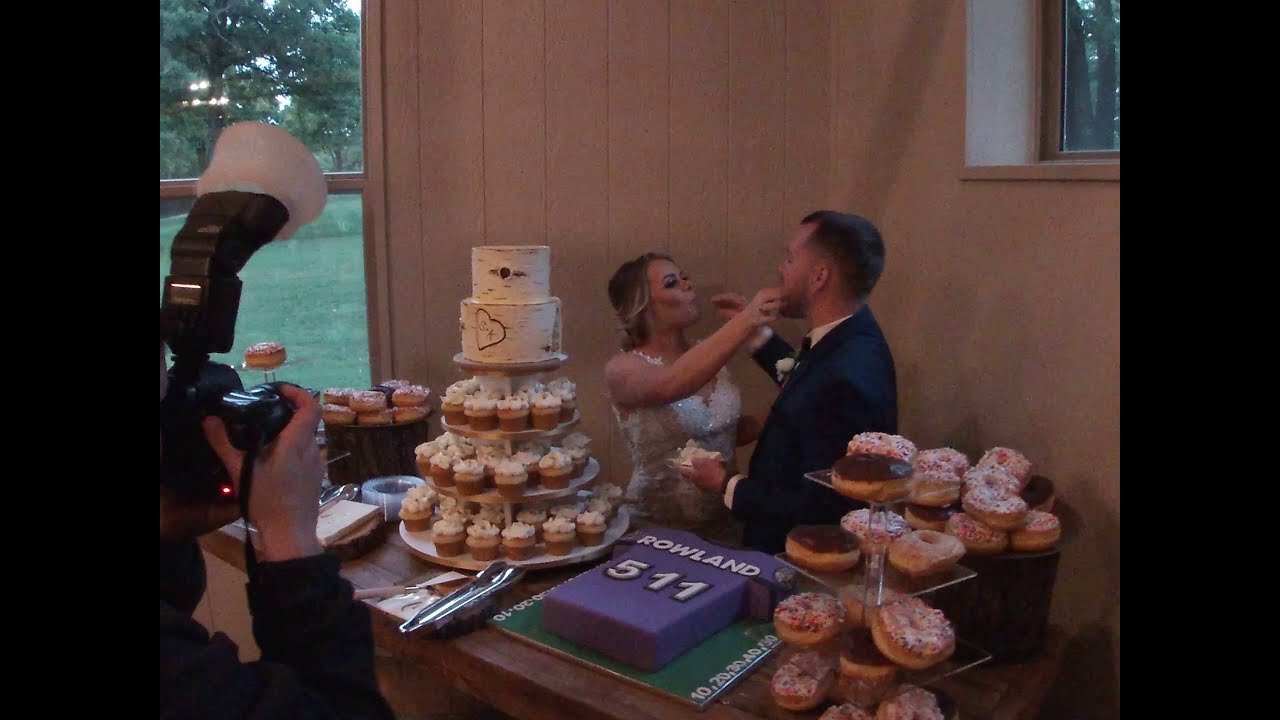This color photograph, oriented in landscape, captures a candid moment at a wedding reception set inside a room with white paneling and windows revealing green grass and trees outside. The bride and groom, of Caucasian descent, are the central figures. The bride, on the left, has brown hair with blonde highlights pulled back, and she is wearing a sleeveless white wedding dress with a V-neck bodice. She reaches towards her groom with her right arm, feeding him a piece of cake. The groom faces her, dressed in a black suit and tie, with a white corsage pinned to his jacket. He holds a piece of cake in his left hand and feeds his bride with his right. They stand behind a wooden countertop that displays a variety of desserts. Notably, there is a purple sports-themed cake shaped like a football jersey inscribed with "Roland 511" in white print, surrounded by a tiered stand of vanilla cupcakes and colorful donuts. A photographer is visible in the lower left corner, capturing this cherished moment. The scene is lit with a subtle, dim ambiance, suggesting it might be evening.